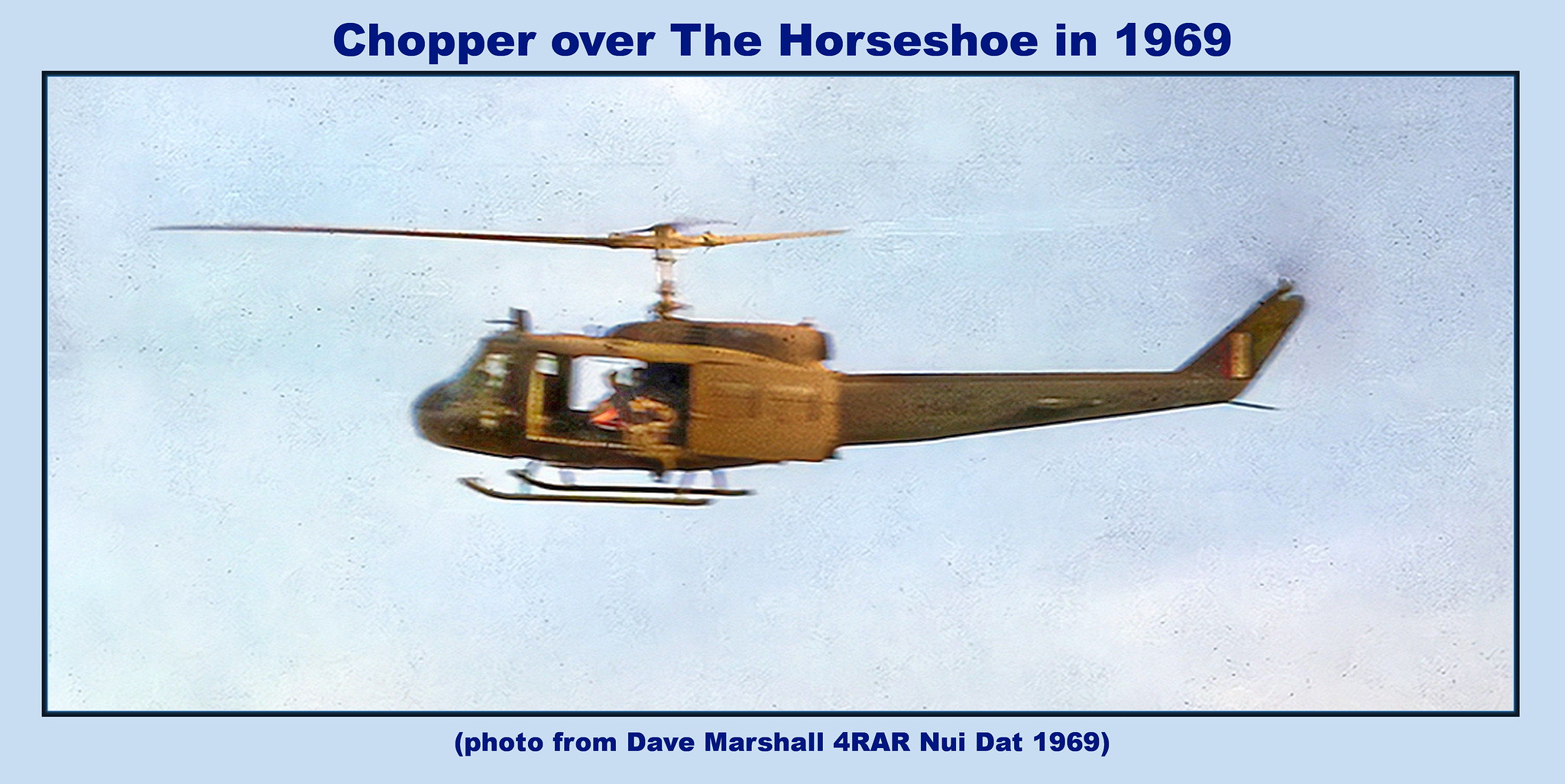This is a landscape-oriented photograph of a vintage brown and green military helicopter in flight during the daytime, surrounded by a blue border. The image is somewhat blurry due to the motion of the helicopter and the spinning main and tail rotors. The sky forms a cloudy backdrop to the helicopter. The helicopter, open on both sides with its sliding doors wide open, reveals glimpses of people or cargo near the openings. 

The photograph is captioned with dark blue text that reads "Chopper over the Horseshoe in 1969" at the top, and at the bottom, in parentheses, "photo from Dave Marshall for RAR Nui Dat, 1969." The helicopter also features a red, white, and blue logo towards its rear. The entire photo has a vintage look, reminiscent of the 1960s, possibly relating to the Vietnam War era.